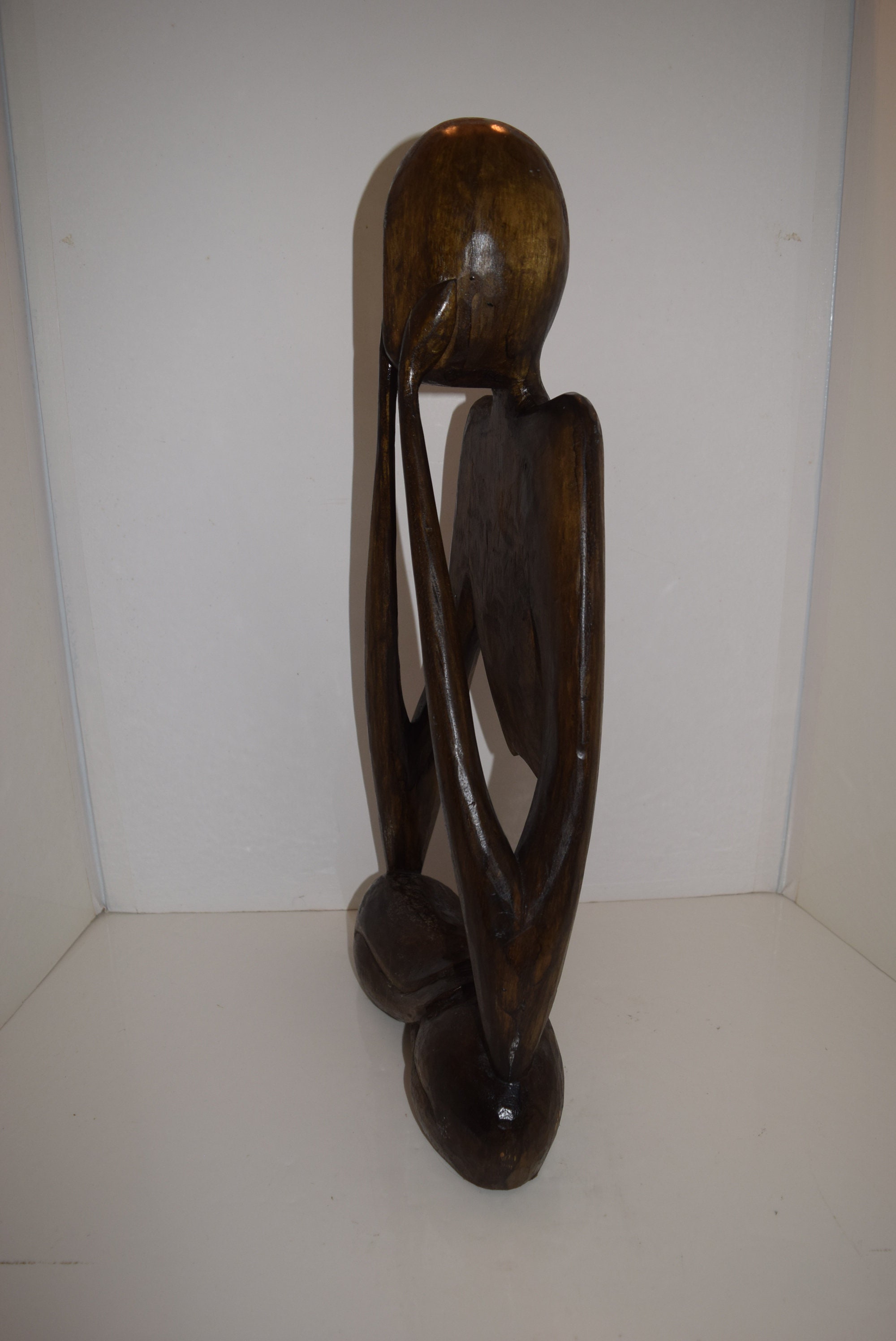This image showcases a small, intricately carved wooden statue housed within a close-fitting, white box. The statue, a deep dark brown in color with a glossy sheen, rests centrally and is partially surrounded by the box’s interior walls, visible on the left, right, back, and bottom. The statue itself resembles a faceless, bald figure with a rounded head and a slender neck, its body flat with extremely elongated arms that extend downwards before bending at sharp angles to place its hands on its cheeks. The lower body is absent, with the elbows resting on what appear to be two egg-shaped objects, similarly dark brown. The overall silhouette of the statue, which could be about 12 inches long, evokes the impression of a yoga pose or a decorative object, with the arms and position suggesting both a sense of concentration and elegance.